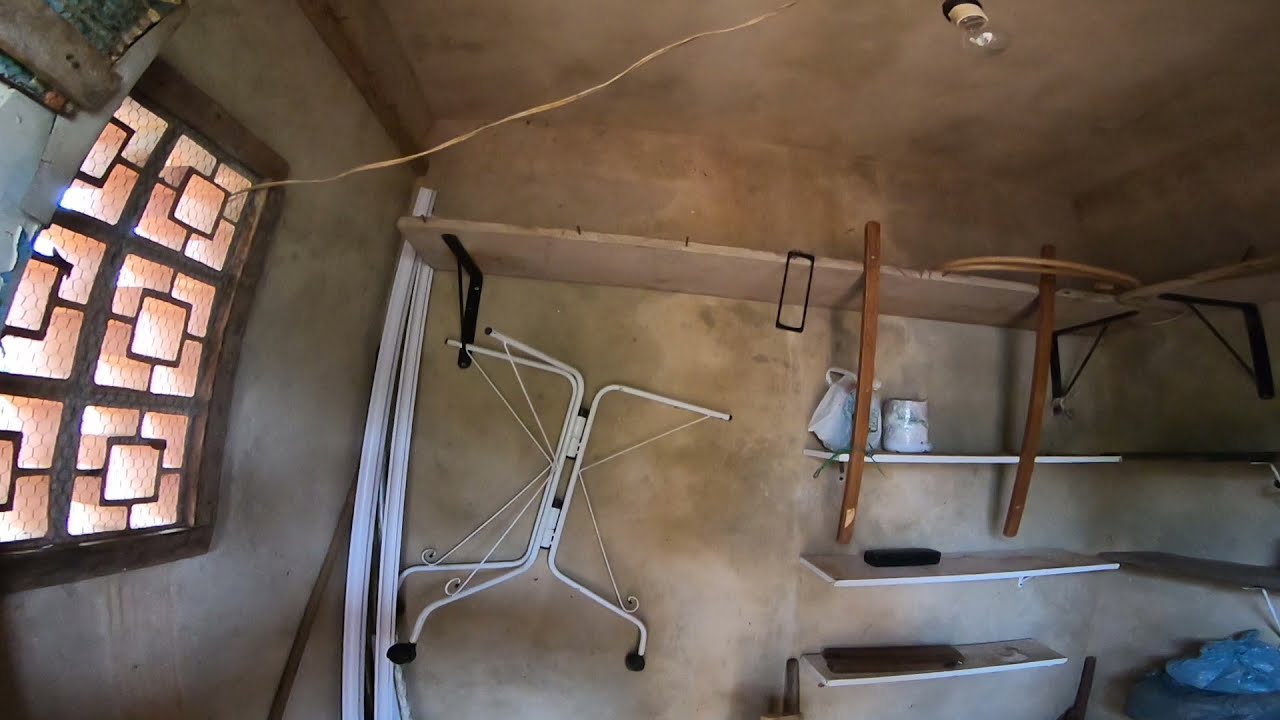The photograph captures the interior of what appears to be a garage or utility room with off-white, clay-like walls. The focal point is a window on the left, featuring a six-panel, wooden frame with orange-tinted glass, making it difficult to see through. A cord runs from the ceiling to the window and is affixed to an exposed light bulb that hangs from the ceiling without a lampshade. 

On the back wall, there are multiple shelves: three white ones holding various items, including a couple of pots, and a white metal contraption resembling a three-wheeled cart hanging from one of the shelves. To the right, a series of four brown shelves contain various items, including something blue on the bottom shelf. The room also contains several vertical poles and brown sticks attached to the walls, adding to the cluttered appearance. The main colors in the room are brown, white, and a hint of orange from the window.